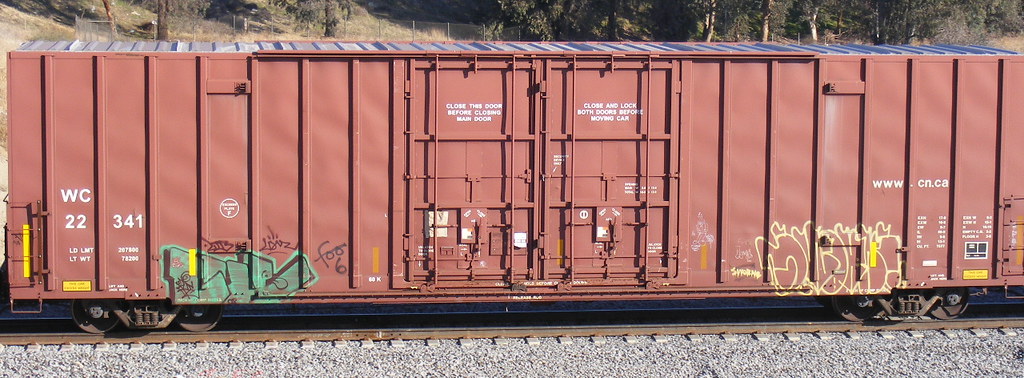This detailed color photograph features a lengthy train car, primarily appearing chocolate brown or possibly a dirty red due to the bright sunlight's effect on its color. The car is stationed on a track surrounded by gray gravel, with some trees and vegetation visible in the background. At the center of the train car, large double doors are present, bearing several white text instructions: "Close this door before closing main door" at the top, and "Close and lock both doors before moving car" on the right side. 

On the left side of the car, in white text, it reads "WC-22, LD-LMT, LT-WT," and nearby, there's additional text with numbers: "341-287-900, T-82-90". A white circle logo is also visible among these markings. The car exhibits various graffiti: green graffiti on the lower left, some yellow graffiti on the right side that includes big letters resembling cartoon characters, and additional cursive graffiti that includes the readable, black text "F-006". On the far right side of the car, the web address "WW.CN.CA" is written in white text, alongside other smaller, unreadable white text. The top of the train car appears gray with blue stripes across it, contributing further to the colorful and vivid detail captured in the bright, sunny scene.